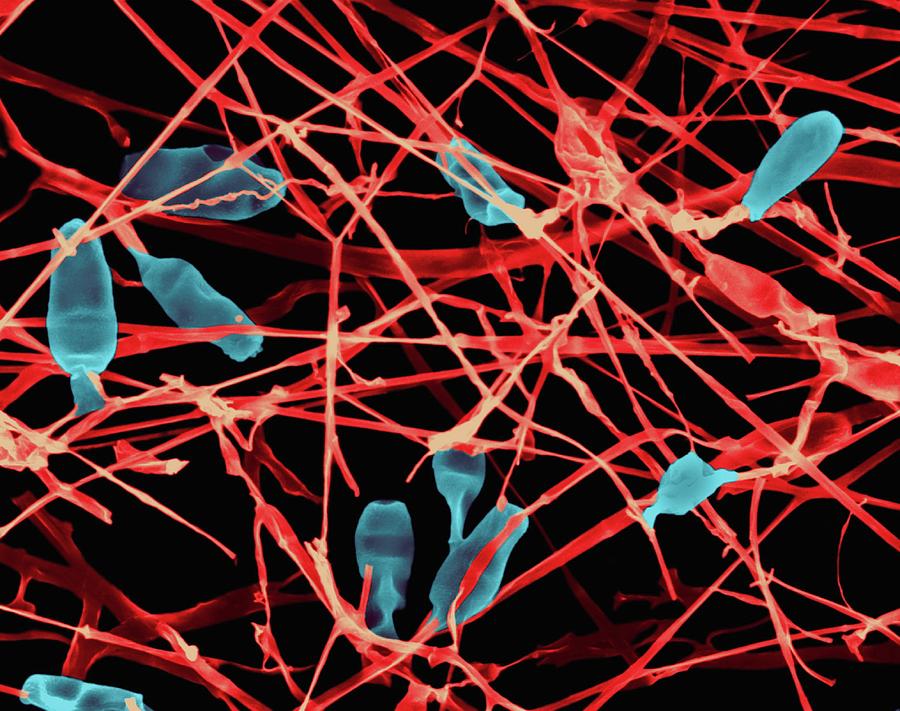This is a highly detailed microscopic image, possibly from an electron microscope, showcasing a network of illuminated fibers and structures against a pitch-black background. The main feature is a chaotic lattice of crisscrossing red and gold lines, resembling tendons or veins, which form thicker clusters at various points. Attached to these fibers are lighter-colored extensions adding to the complexity. Scattered throughout the image are translucent, blue, oblong structures that resemble balloons or bacterial shapes, with their glowing appearance suggesting a neon illumination, typical of certain microscopy techniques. Specifically, there are around ten of these blue bodies, concentrated mainly in the upper left and middle sections of the image, with a few spread out towards the bottom and right. The overall scene is both abstract and alien in its intricate detail and chaotic arrangement.